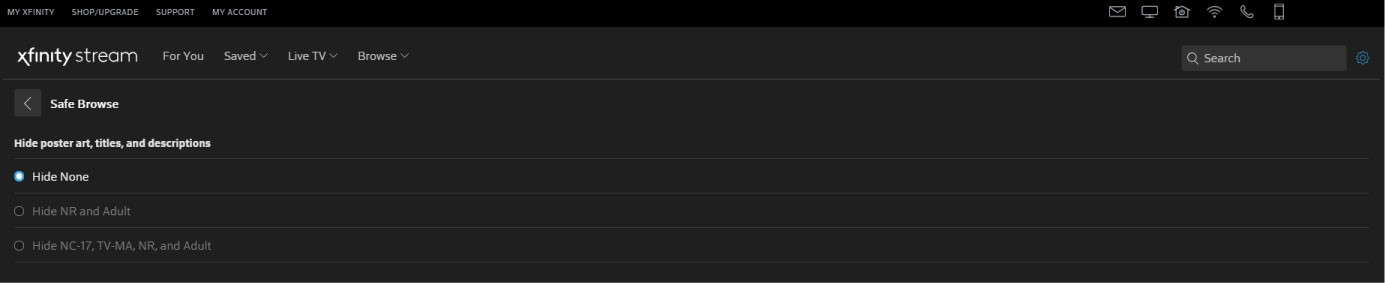The image depicts a detailed interface of Xfinity Stream settings. The interface is presented in a dark, horizontal rectangular box with small, intricate text. At the top, a sleek black strip contains the navigational options: "MyXfinity," "Shop/Upgrade," "Support," and "My Account," all in grey. To the far right of this strip, a series of icons are aligned, representing Mail, a Monitor, a Home, a fully-filled WiFi signal, a Phone, a Phone handset, and a Mobile phone.

Below, in lighter grey text, it reads "Xfinity Stream," indicating that this interface is part of Xfinity's services, which include cell phone, internet, and cable services. Further classifications are listed below: "For You," "Saved," "Live TV," and "Browse," each accompanied by a downward-facing drop-down arrow. Underneath, the option "Safe Browse" is highlighted in white within a light grey box featuring a left-pointing arrow. 

Additional settings include options to hide poster art, titles, and descriptions, alongside visibility settings labeled "Hide None," marked by a white dot inside a blue circle, indicating the choice not to hide any content. The other options not selected are in muted grey: "Hide NR and Adult" and "Hide NC-17, TVMA, NR, and Adult."

To the right of these settings is a light grey search bar containing a search icon, and adjacent to it, an outlined gear icon in blue signifies additional settings. This meticulous interface belongs to the Xfinity Stream service, showcasing various settings options available to users for content management and customization.